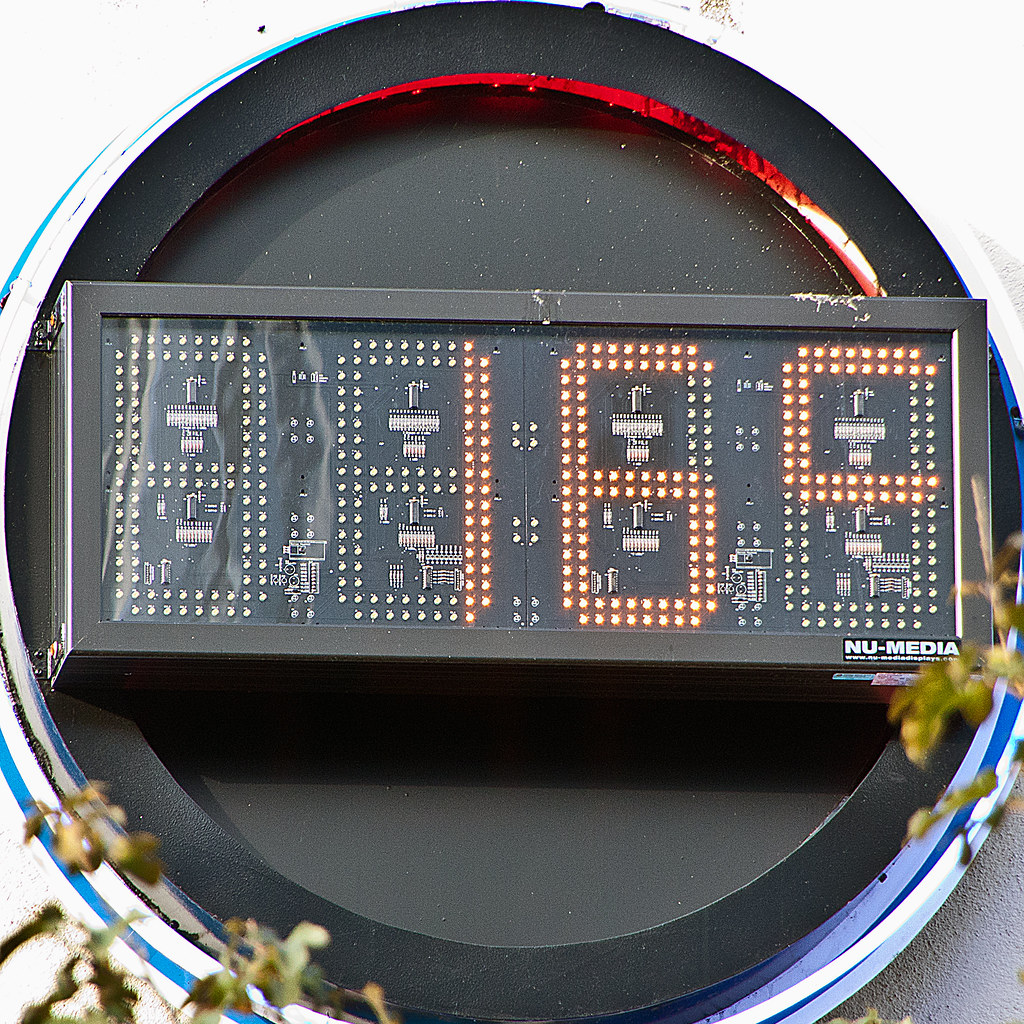The photograph features a close-up view of a digital readout, possibly of a thermostat or thermometer, housed in a black circular frame. The lower portion of the frame is accentuated with blue and white coloring, while the upper portion displays red and white coloring. In the bottom right-hand corner of the frame, there's a distinctive rectangular black section with the text "New Media NU-MEDIA" inscribed in white letters. The display shows intricate details of its internal circuitry, revealing the configuration of LED lights that could illuminate numbers. Currently, the readout indicates a temperature of 16°C, with the characters "1 6 C" clearly visible.